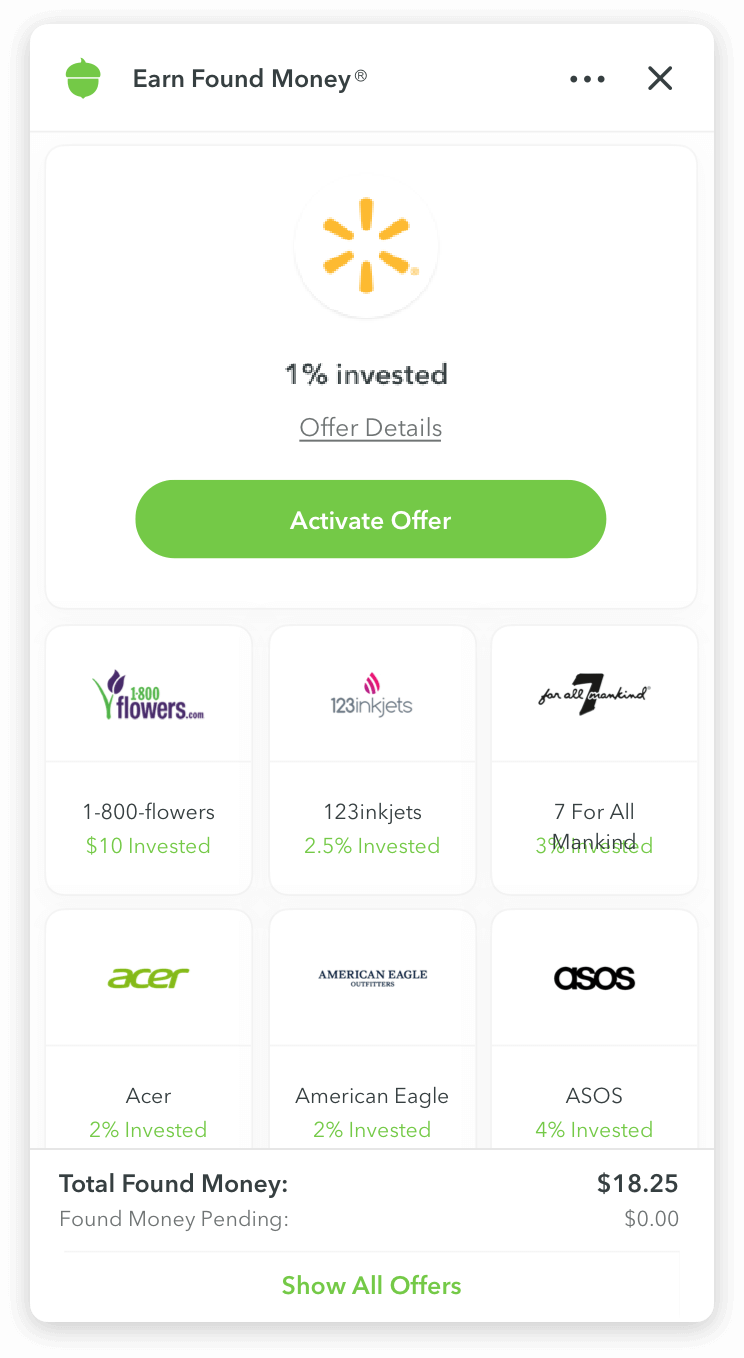A tall, rectangular screenshot appears to be from a cell phone and shows an interface of the Acorn app. In the upper left-hand corner, there's a distinctive acorn logo, followed by the text, "Earn Found Money." Adjacent to this text, three black dots are arranged horizontally, and a prominent 'X' icon on the right allows users to close the screen.

Dominating the center of the page is the Walmart logo with a note indicating "1% invested." Beneath it, there is a green, oval-shaped button labeled "Activate Offer." The page further showcases two rows of investment options, each featuring the logo and details of different retailers. Among the options are:

- 1-800-Flowers.com: $10 invested
- 1-2-3-Ink-Jets: 2.5% invested
- 7 For All Mankind: 3% invested
- Acer: 2% invested
- American Eagle: 2% invested
- ASOS: 4% invested

At the bottom of the screen, it indicates the total "Found Money" amounts to $18.25, with "Found Money Pending" listed as zero.